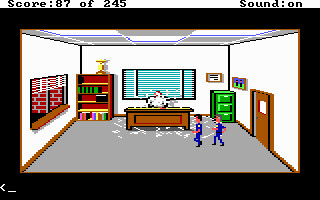In this vibrant, pixelated scene reminiscent of an early 90s computer game, an office setting is vividly depicted with colorful, retro-style graphics. At the top of the screen, a score displayed as "87 of 245" is flanked by an indicator reading "Sound On" to the right. On the left side of the office, a bookcase adorned with a trophy occupies the space beneath an open-blinded window, allowing light to spill into the room. Another window behind the centrally-placed desk is obscured by closed blinds, creating a contrast in lighting.

The desk itself is cluttered with scattered papers, presenting a chaotic workspace. Seated at the desk is a pixelated character, seemingly engrossed in their tasks amidst the disarray. To the right, a door is prominently featured, through which two characters garbed in blue outfits are walking in, possibly signaling the arrival of colleagues or visitors. The meticulous attention to detail in this office tableau effectively captures the nostalgic essence of classic video game design, transporting viewers back to the golden era of early computer animation.